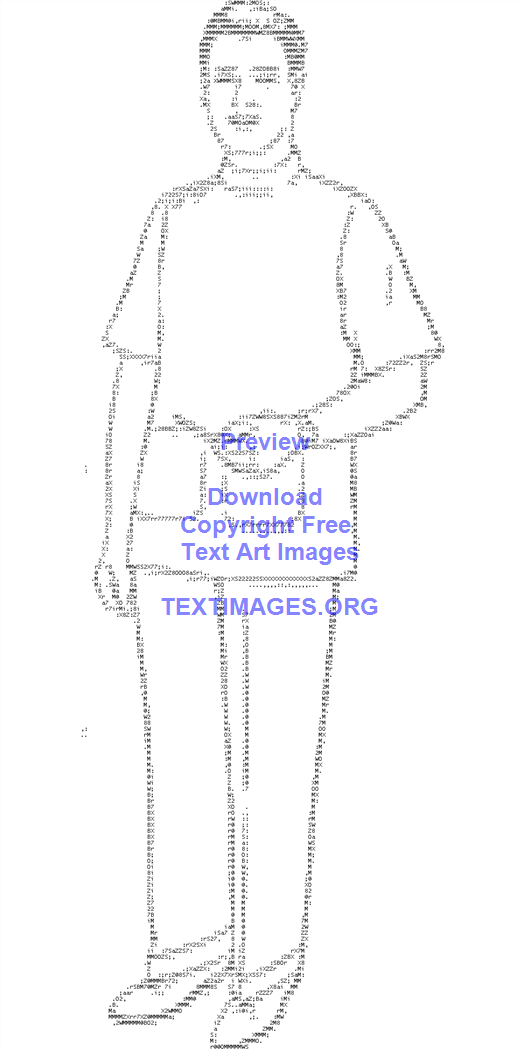This digital artwork, distinctly crafted using text and keyboard symbols, features a detailed silhouette of a man that dominates the entire image. The man, depicted with black hair, a clean-shaven face, and a smile, wears a short-sleeve shirt possibly with front pockets, long trousers, shoes, and a wristwatch. His right hand hangs down while his left hand is raised, holding an unidentified object. The color palette includes shades of white, black, gray, and purple, though the artwork lacks any borders or frames, set against a white background. The style and setting suggest it is an advertisement for a text art image website, with a watermark text in the center of the image reading "Preview, Download Copyright-Free Text Art Images, textimages.org," partly overlaying the man's abdomen and pelvis area.